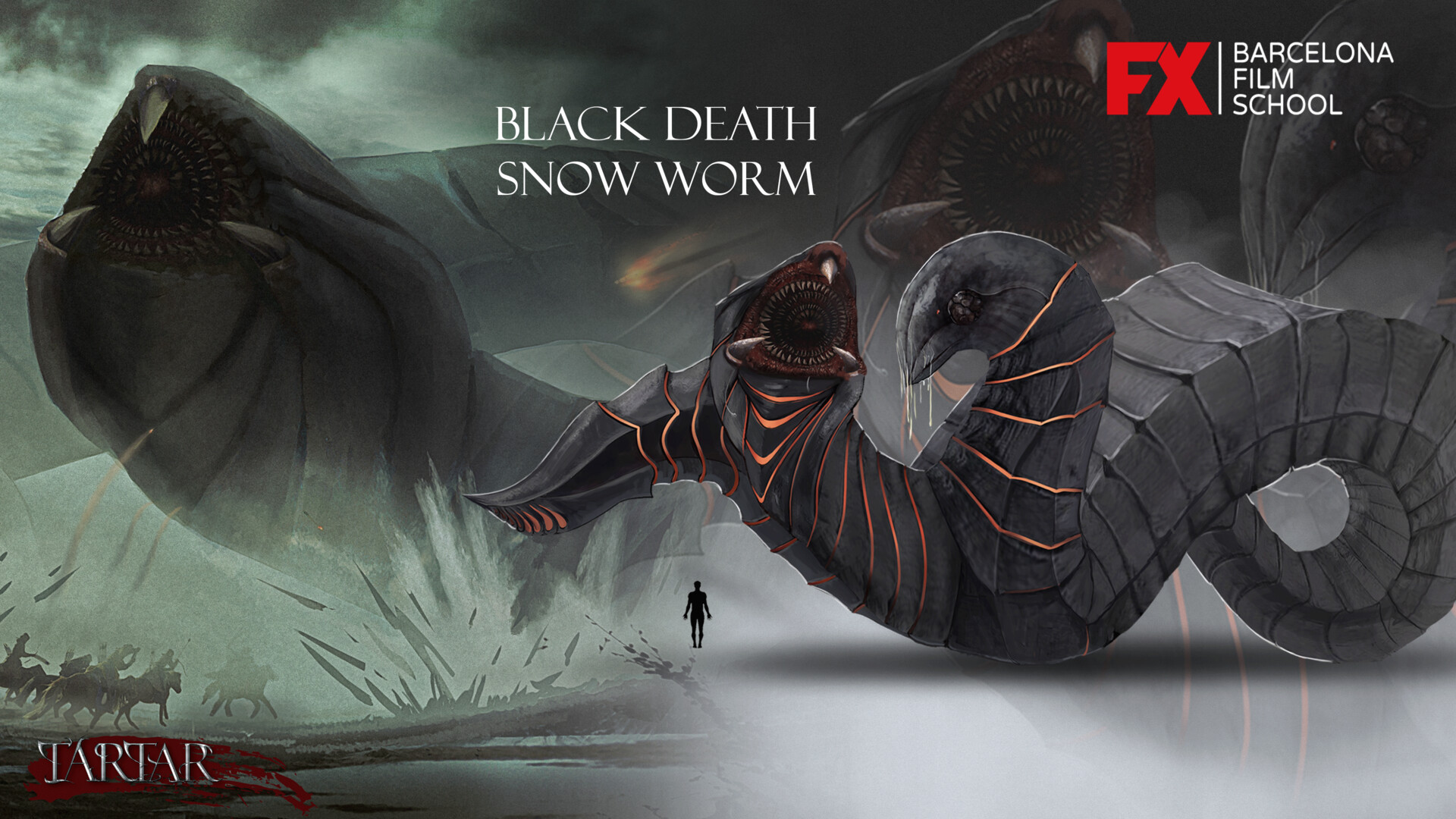In this computer-generated concept art poster for a movie or show titled "Black Death Snow Worm," prominently displayed in the top middle in white text, we see a terrifying and detailed illustration of a menacing creature. The top right corner features the red letters "FX" followed by a thin vertical white line, under which "Barcelona Film School" is written in white. In the bottom left corner, the word "Tartar" is presented in a medieval font over a blood smear, emphasizing the horror theme.

The monstrous "Black Death Snow Worm" spans the left side, presenting a chilling visage reminiscent of the Sarlacc from "Star Wars" or the Shai-Hulud from "Dune." It features a triangular head with one mouth detailed in vivid close-up, showcasing three prominent fangs arranged in a triangular fashion along with rows upon rows of sharp teeth inside. The worm's multiple heads give it a hydra-like appearance, with one open-mouthed head centrally visible and another closed-mouth head on the right. The leftmost appendage is vague, barely resembling a head.

The creature's body is adorned with long, rectangular, rigid scales interlaced with fiery red or orange lines, adding a dynamic sense of movement and menace. The creature even exudes an aura of wetness, with short tentacle-like appendages dripping a viscous liquid, potentially saliva, intended to underscore its chilling lethality.

In the bottom center of the image, a black silhouette of a human figure provides a scale reference to the worm's immense size, adding to the ominous atmosphere. The background is dark and clouded, enhancing the overall sense of dread, possibly augmented by the shadowed figures of horses and their riders in the distance, further deepening the poster's nightmarish scene.